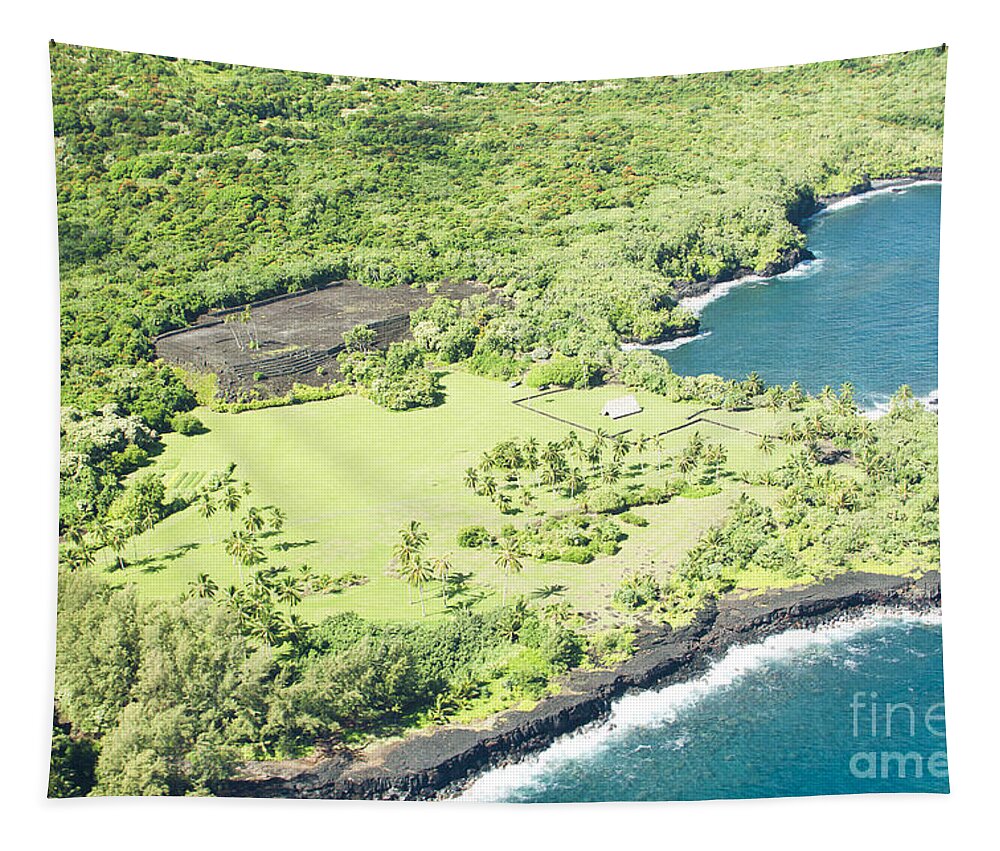This vivid aerial photograph captures a stunning tropical coastline bathed in bright sunlight. The coastline is lined with jagged rocky cliffs that stand against the crashing waves of the deep blue ocean, visible in both the lower and upper right corners of the image. Lush greenery dominates the scenery, with numerous palm trees and other dark green vegetation covering much of the land. An open grassy area stretches alongside the cliffs, offering a stark contrast to the rugged rocks.

In the background, towards the upper left corner, there is a cleared, level expanse of brown dirt, punctuated by a few scattered palm trees. This appears to be a raised plot, possibly prepared for future construction. Centrally located, slightly off to the right, stands a small white tent, adding a solitary man-made element to the natural landscape. There are no visible people or additional structures, emphasizing the untouched and serene beauty of this tropical paradise. The overall scene suggests a remote island, possibly in the Philippines or another equatorial region.